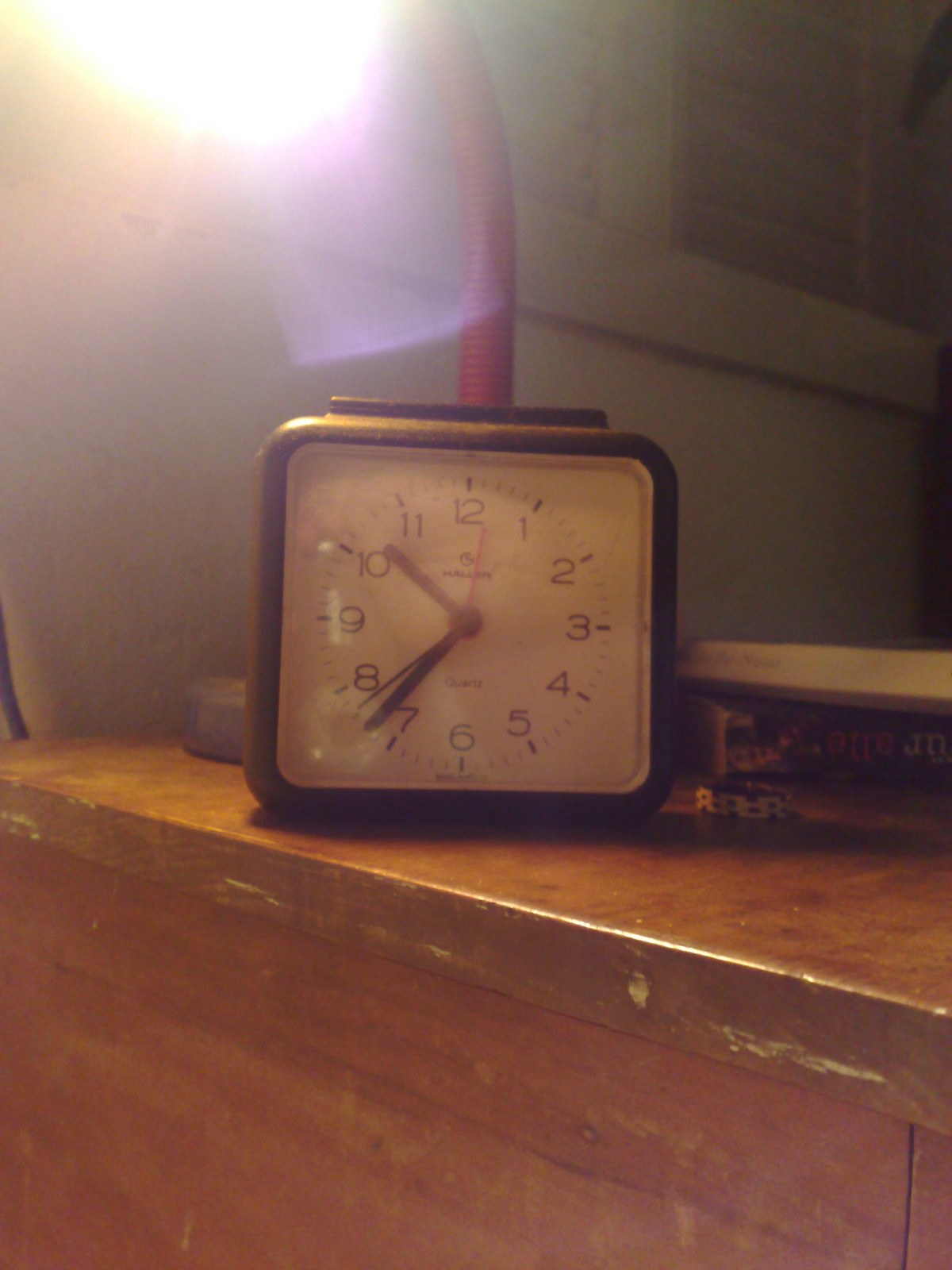The image depicts a dated bedroom setting with a prominent focus on a square analog alarm clock, showing the time as approximately 10:42 PM. The clock has a white face with black hour and minute hands, a red second hand, and an additional button on top, likely serving as a snooze function. Resting on an old, battered, light brown pine nightstand with visible paint marks and scratches, the clock is accompanied by various indistinguishable items, possibly books or binders. Behind the clock, there is a thin-framed mirror and a red, gooseneck desk lamp emitting a soft yellow light that glares out part of the scene. The backdrop includes white walls and potential blinds, contributing to the vintage ambiance reminiscent of the 1970s or 1980s.